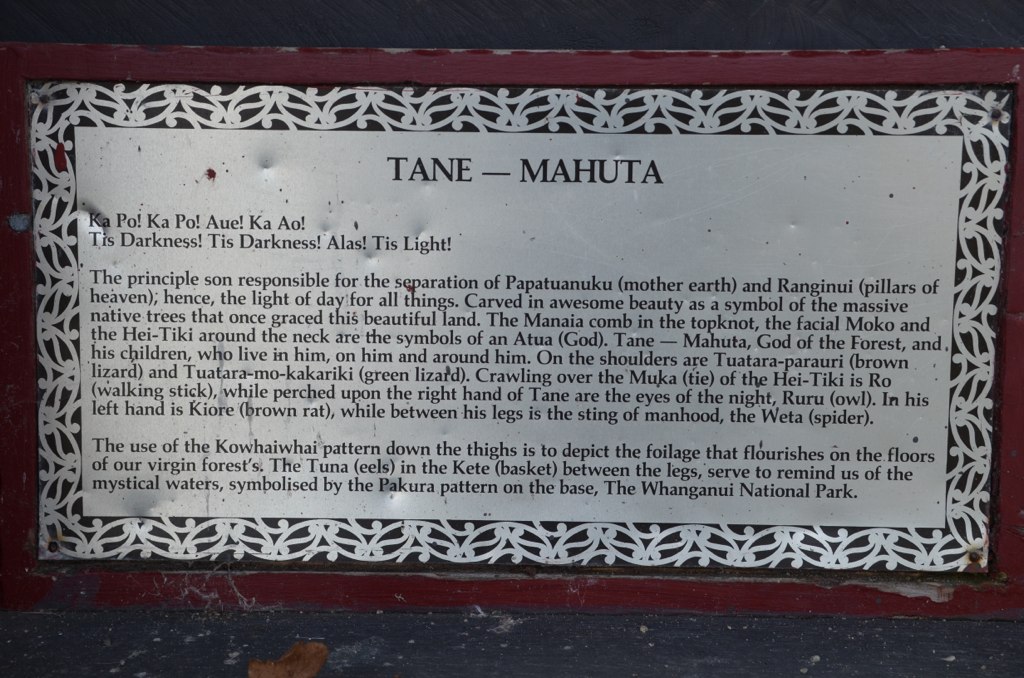The image depicts a close-up photo of a framed sign, slightly leaning against a grayish-black, chipped wall. The frame of the sign is made of red wood, while the central area consists of a light silver metal background embedded with black text. The sign has ornate filigree details on the sides, and shows signs of wear with a couple of dents. 

At the top, the text reads "Tane Mahuta" (T-A-N-E dash M-A-H-U-T-A), followed underneath by smaller text "Kapu Kapu Ah Kapu, Tis Darkness, Tis Darkness, Alas Tis Light." Further down, the main body of the text elaborates on the mythology, naming Tane Mahuta as the principal son responsible for the separation of Papatuanuku (Mother Earth) and Ranginui (Pillars of Heaven), leading to the creation of daylight. 

The sign also describes the symbolic carvings representing native trees and associated deities. It mentions the Makama comb in the top knot, facial moko, and high tiki around the neck symbolizing the Atua god Tane Mahuta, god of the forests, along with his children. Specific creatures like Tarahuta (Brown Lizard) and Terutama Karakiriki (Green Lizard) are noted on the shoulders, while Ro (Walking Stick) is depicted crawling over the high tiki. Additionally, the right hand features Ruru (Owl), the left holds Kahur (Brown Rat), and between the legs is Wepta Spider. The text further narrates the depictions of foliage and mystical waters through patterns and carvings down to the base.

The content concludes by referencing the Whanganui National Park, underscoring the cultural and natural heritage symbolized by the sign.